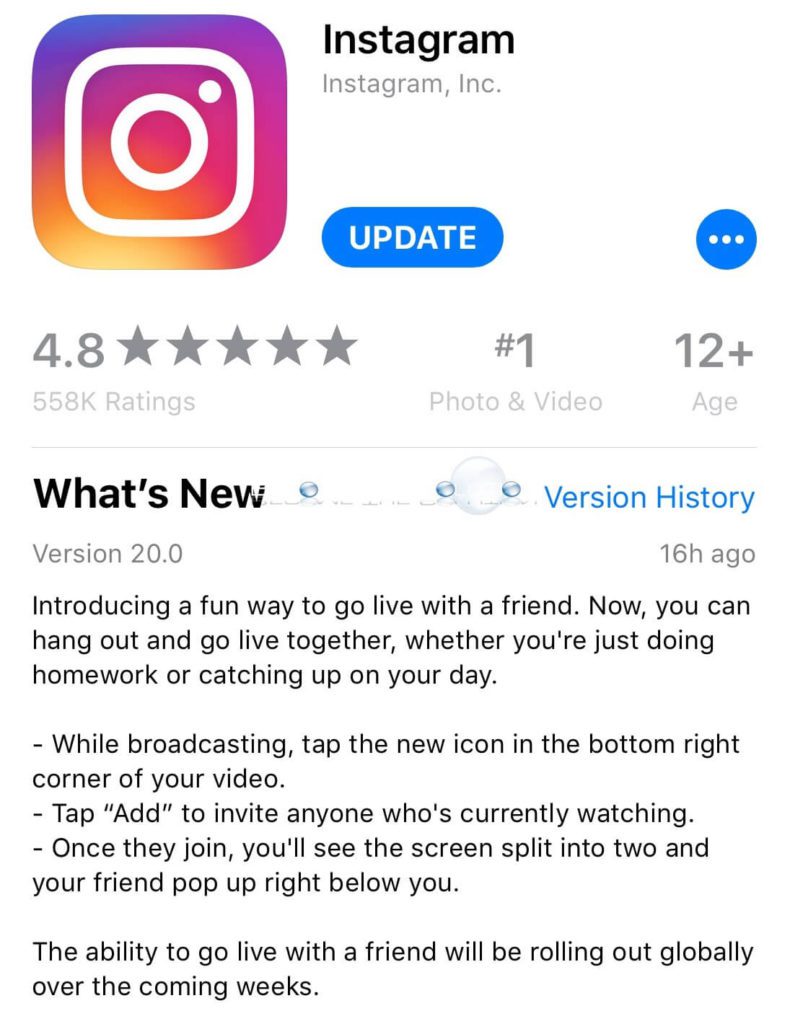The image is a detailed screenshot of the Instagram app update page on a mobile device. On the left-hand side, there's the Instagram icon, showcasing the familiar gradient logo with a blend of purples on the top, transitioning to pinks on the right side, oranges on the left, and yellows at the bottom. The icon is a vertical rectangle with rounded corners. Inside the gradient background, a white outline mimics the outer shape, containing a white circle with a small white dot in the upper right corner.

Next to the icon, "Instagram" is written in bold black letters, followed by "Instagram, Inc." in gray underneath. Directly below, there's a blue oval button with white capital letters reading "UPDATE." To the right of the update button, there is a blue circle containing three horizontal white dots.

Further down, in gray text, it reads "4.8" accompanied by five fully colored gray stars, indicating user ratings. Below this, it states "558K ratings." In the middle column, it lists "No. 1" followed by "Photo & Video," and in the third column, it states "12+" with "Age" underneath.

The section titled "What's New" appears in bold font. On the right side, in blue text, it says "Version History." To the left, it mentions "Version 20.0" in gray and, to the right, "16h ago."

The update description begins by introducing a new feature: "Introducing a fun way to go live with a friend. Now you can hang out and go live together, whether you're just doing homework or catching up on your day." It continues with instructions on how to use the feature: "While broadcasting, tap the new icon in the bottom right corner of your video. Tap 'Add' to invite anyone who's currently watching. Once they join, you'll see the screen split into two and your friend pop up right below you." It concludes by stating that "The ability to go live with a friend will be rolling out globally over the coming weeks."